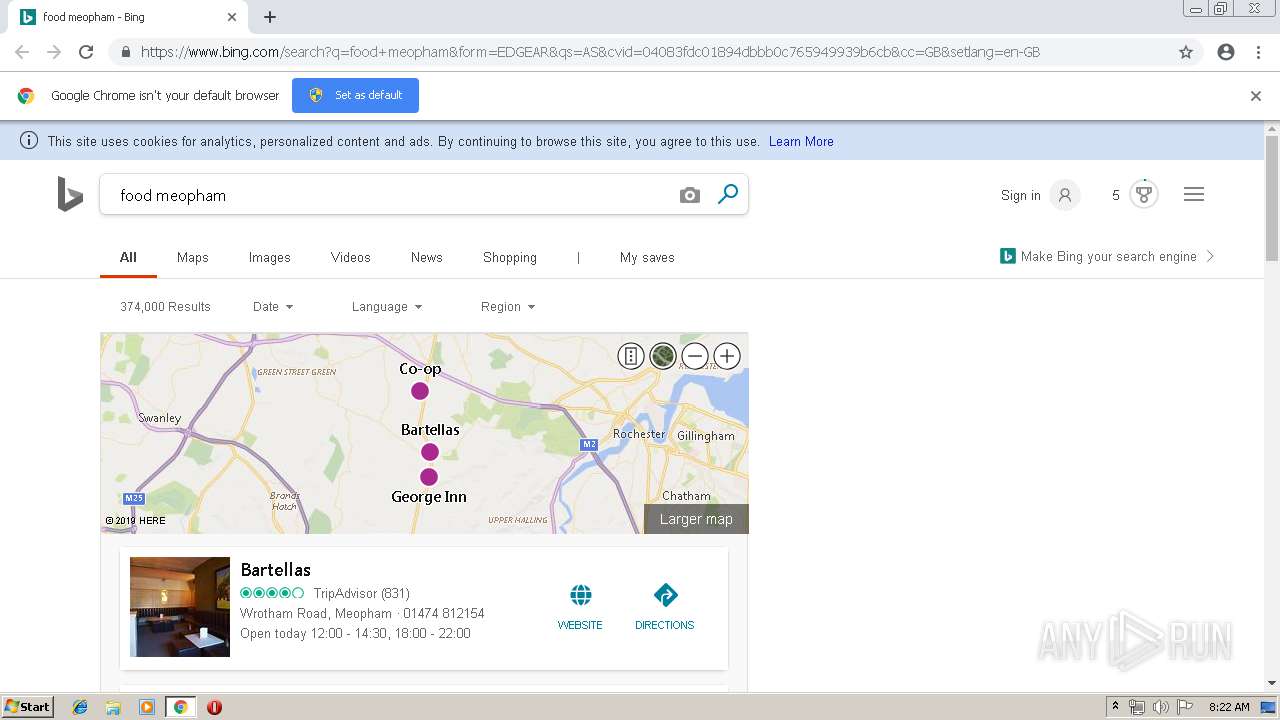The image is a screenshot of an internet browser displaying a Bing search results page. The search query entered is "meal fam." The interface showcases several categories of results at the top, including All, Maps, Images, Videos, News, and Shopping, with the 'All' category currently selected.

Just below the search categories, a highlighted map features the location of "Bartella's," presumed to be a restaurant. The map provides today's operating hours, the address at Rotham Road, Meal Fam, and options to visit the restaurant's website or obtain directions.